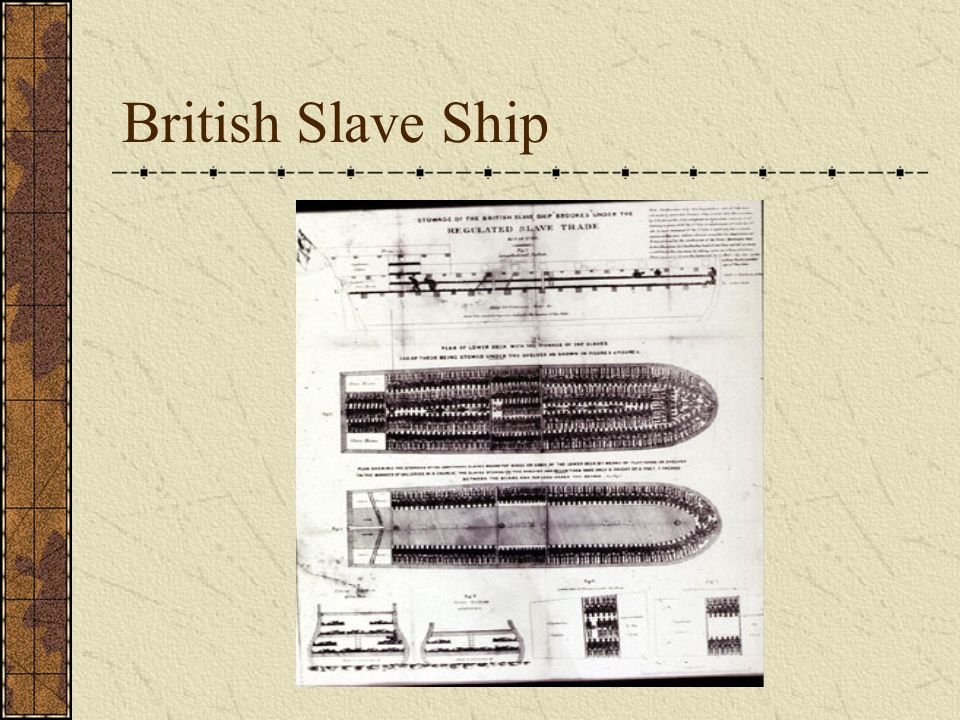This image appears to be an illustrative page from an old textbook or possibly a rendering of a historic document focused on the British slave trade. The background is an off-white or beige color, giving it an aged look. Along the left edge is a vertical brown stripe that resembles the book binding. At the top left, in brown text, it reads "British Slave Ship." 

In the center of the image, slightly off-centered and crooked, is a detailed black-and-white diagram of a British slave ship. This diagram is enclosed in a white rectangular box, standing out against the beige background. The ship is depicted from both an exterior perspective and a cross-sectional view, showing the interior layout across two levels. The lower section of the diagram depicts how enslaved people were constrained in cramped, box-like compartments.

Above the diagram, in slightly blurred text, it reads "Regulated Slave Trade," suggesting the context of the image pertains to the regulations or conditions of the slave trade. Surrounding the diagram, additional text describes the illustration, but it's small and difficult to read clearly. Overall, the color scheme includes shades of tan, brown, black, white, and some gray, and the entire layout mimics a page from an educational slide or presentation on the history of the British slave trade.